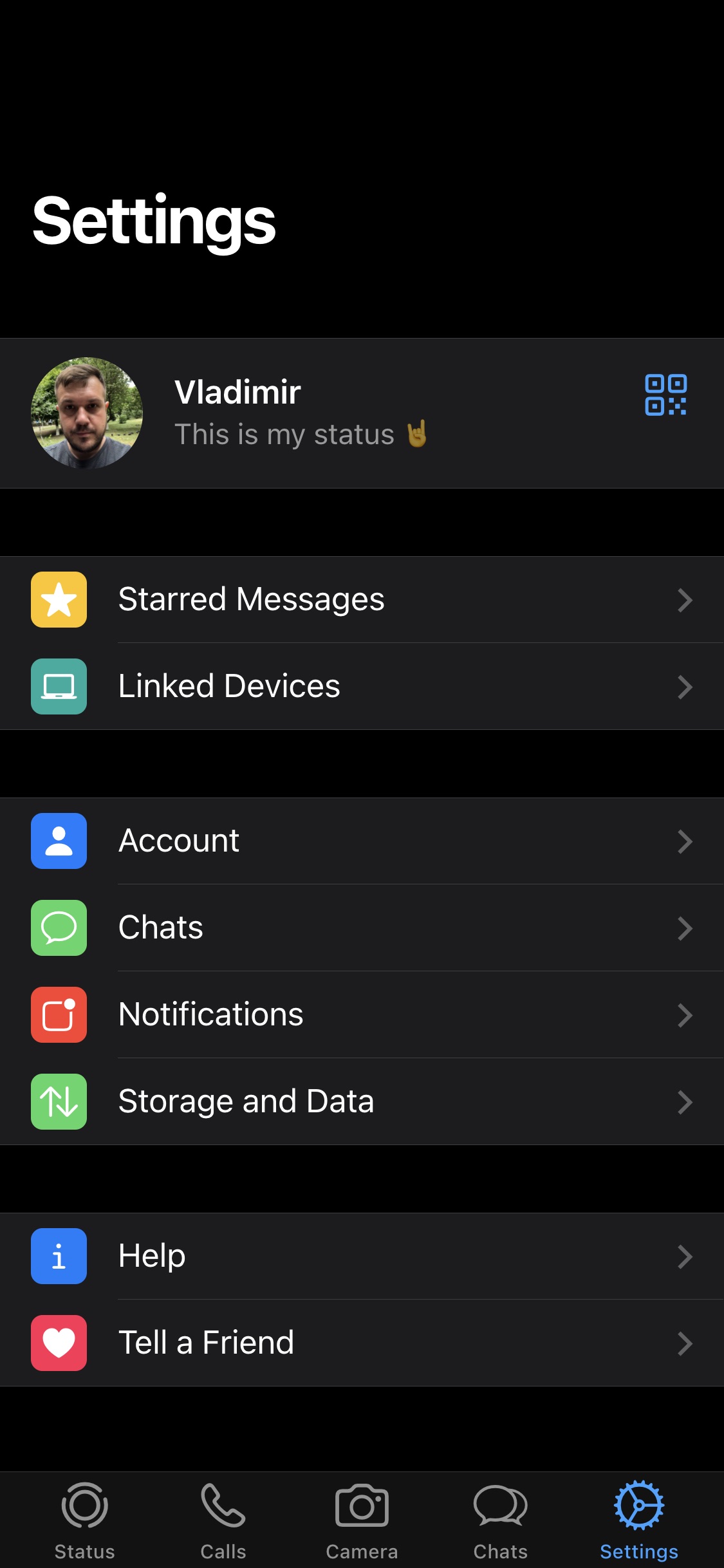The image appears to be a screenshot of Vladimir's WhatsApp profile settings page. At the top, in prominent white block letters, the word "Settings" is displayed. Below it, the name "Vladimir" is shown, accompanied by a profile picture of a white man with approximately three-inch-long hair. The status section next to the profile picture reads "This is my status" and features an emoji with two fingers. Beside the status, there is a QR code intended for sharing the profile.

The screen includes a list of several rows with distinct labels and corresponding icons:
- "Starred Messages" 
- "Linked Devices" (icon: a laptop)
- "Account" (icon: a profile)
- "Chats" (icon: speech bubbles)
- "Notifications" 
- "Storage and Data"
- "Help" (icon: an information 'i')
- "Tell a Friend" (icon: a heart)

At the bottom, there are navigation options with accompanying icons:
- "Status" (icon: a circular status symbol)
- "Calls" (icon: a phone)
- "Camera" (icon: a camera)
- "Chats" (icon: speech bubbles)
- "Settings" (icon: a cogwheel)